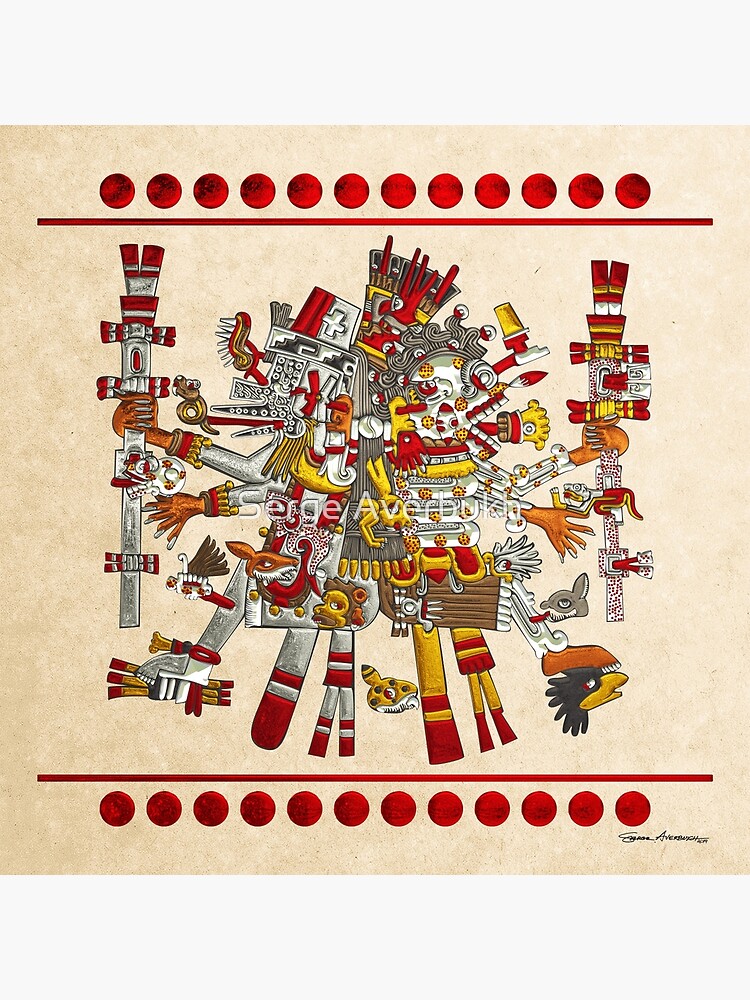The image is a highly intricate and complex artistic creation, characterized by a vivid and dynamic use of colors, primarily red, yellow, silver, and bronze, set against a beige background. Dominating the composition is a central figure that seems to be an amalgamation of various elements reminiscent of totem pole creatures, featuring multiple animal heads such as a rabbit, bird, and fox, alongside numerous human hands and arms. This figure exudes a sense of both chaos and unity, as it holds silver sticks and swords adorned with red and yellow accents.

At the top and bottom of the image, a line of red circles is framed by horizontal red lines, creating a mirrored border that encapsulates the central figure. The art evokes a blend of cultural influences, drawing comparisons to Japanese, Maori, and Native American aesthetics. The detailed depiction includes myriad squiggly lines and elaborate designs, with what appears to be an artist's signature located at the bottom right. The entire composition is a vivid, colorful tableau that captures a sense of intricate symbolism and artistic prowess.